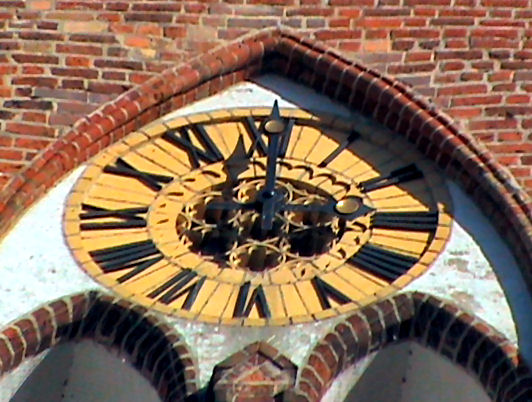The image captures the face of a clock embedded in the exterior wall of a brick building. The building features a variety of red brick shades, adding texture and depth to its façade. The clock is set in a recessed, white plastered, arched alcove that offers a striking contrast to the surrounding bricks. The clock face itself is yellow, adorned with black Roman numerals for legibility. 

The clock has both a minute and an hour hand, each rendered in black with a gold circle at the pivot point. At the center of the clock face, where the hands meet, is a circle of rosettes adding a decorative touch. Below the clock, the building features two additional arched recesses, further enhancing its architectural interest and giving the clock a commanding presence on the wall.